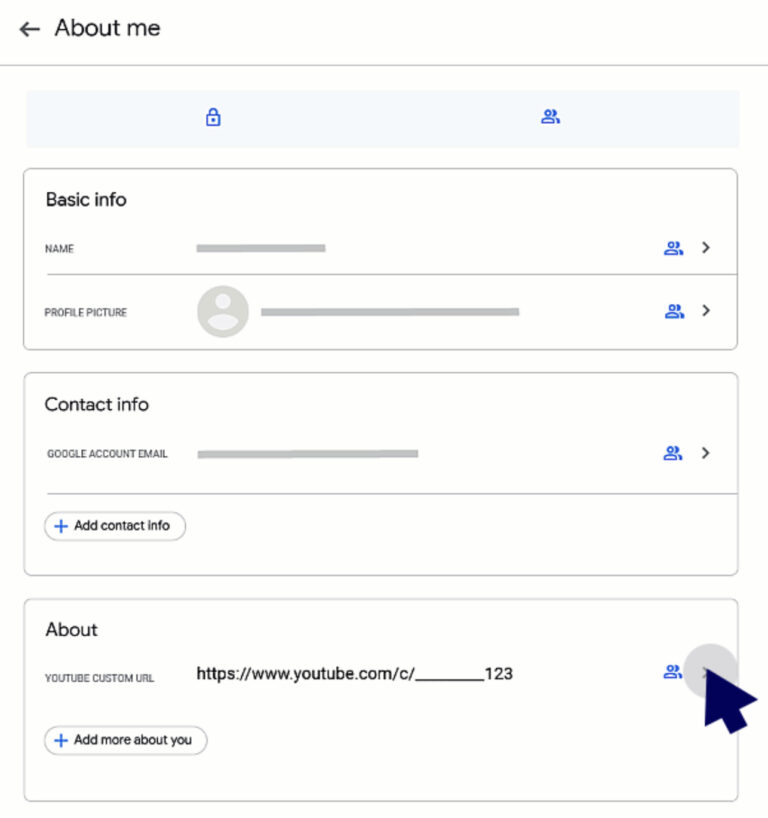The image depicts a computer or phone screen showcasing a digital design page, potentially from an app or website. At the very top, the page is titled "About Me" in black text with an arrow pointing to the left, followed by a gray header line. Beneath this, there is a faint bluish-gray box containing two blue icons: a lock on the left and a person with a person behind them on the right.

Below this, there is another section labeled "Basic Info" in bold font. It includes "Name" accompanied by a gray bar, a blue icon of two people, and a right-pointing arrow. A dividing line separates this from the "Profile Picture" section, which displays a blank gray profile image, another gray bar, the blue people icon, and a right-pointing arrow.

Further down, a gray box titled "Contact Info" in bold font appears. It contains "Google Account Detail" followed by a gray bar, a blue people icon, and a right-pointing arrow. Another gray dividing line leads to a blue plus sign and the text "Add Contact Info".

The final section is a gray box labeled "About You". It displays a custom YouTube URL, "https://www.youtube.com/C/underline123", a blue dot, and a large blue arrow indicating a click action on the right-pointing arrow next to it. Below this, a plus sign with the text "Add More About You" is present.